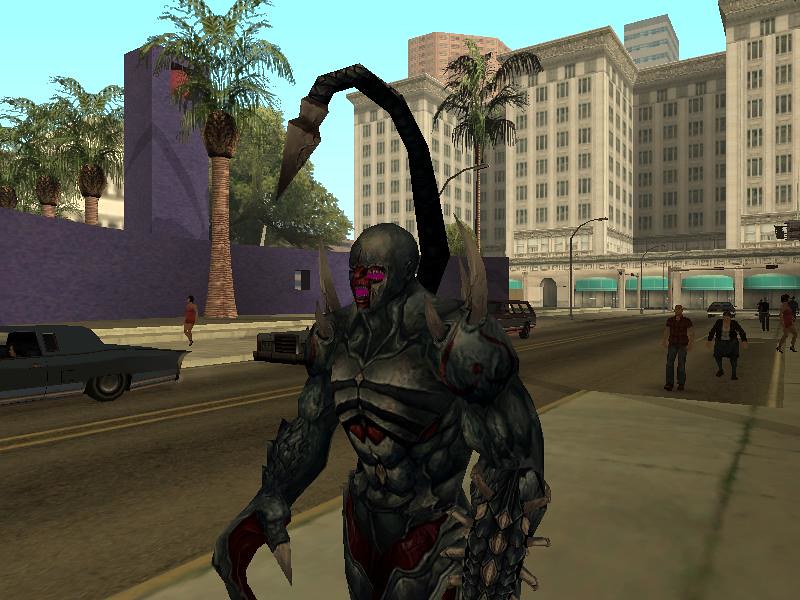In this digitally rendered still image, likely sourced from a video game or artistic creation, the scene unfolds along a city street dominated by a towering multi-story building that could be either a hotel or an apartment complex. The building's facade is punctuated by numerous windows for each unit, while the ground level is lined with green awnings adding a splash of color. The streetscape is alive with pedestrians walking both on the sidewalks and along the street itself, giving a sense of everyday urban bustle. Multiple palm trees can be seen in the background, suggesting a temperate or tropical city setting. However, the central focus of the image is an imposing, monster-like character. This creature is clad in menacing black armor and possesses a face covered with a series of red, hole-like features filled with sharp teeth. Emerging menacingly from its back is a large, scorpion-like stinger, arched overhead and poised downward, adding a sense of imminent threat to this fantastical urban tableau.